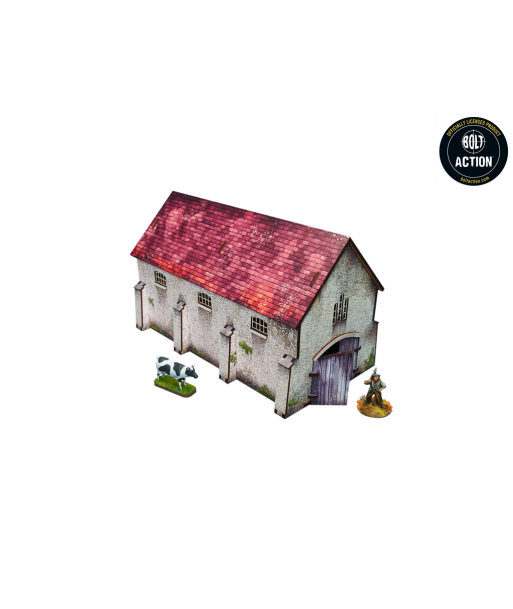The image depicts a detailed ceramic figurine of a gothic-style farmhouse with a red shingled roof. The farmhouse's facade is primarily white stone with distinct gray wooden doors that are slightly open, reminiscent of barn doors. There are three windows visible on the front side, each framed by stone arches extending from the ground. Above the main door, there's an additional window. To the left of the farmhouse, there is a detailed statue of a black and white cow standing on a patch of grass, while to the right, a small figurine of a farmer wearing blue overalls and brown slacks stands on another patch of grass. In the upper right corner of the image, a black circle with white text reads "Bolt Action." The background and flooring surrounding the farmhouse are entirely white, giving it a simplistic, isolated appearance similar to what one might see in a computer or mobile app game.